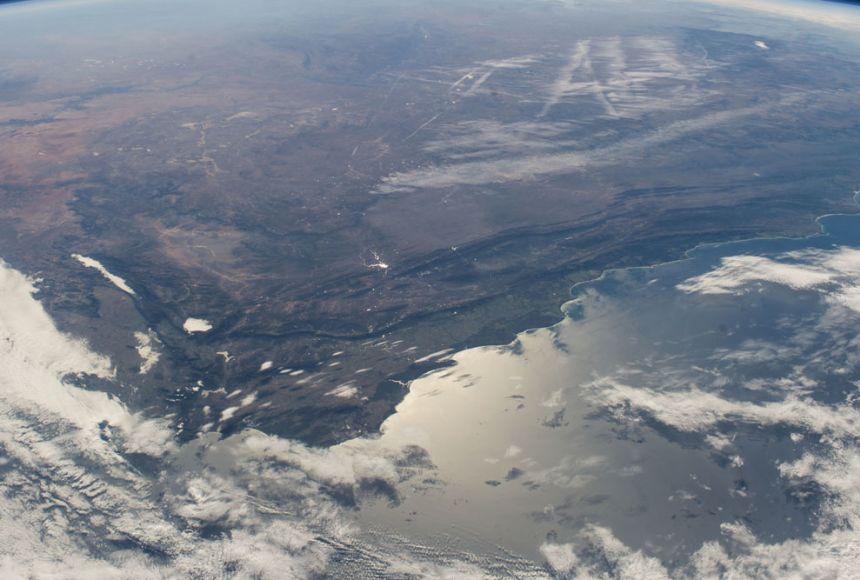This image presents an aerial view of Earth, likely taken from a spacecraft or high-altitude airplane. The photo captures the curvature of the planet, with the edge visible in the upper left and right corners, providing a sense of Earth's roundness. The upper half of the image is dominated by a large landmass characterized by a rocky, rugged terrain that includes cliffs along the shoreline. The land is primarily in shades of gray, black, brown, and green, with a mix of land features such as cliffs.

The distinct land features include small bodies of water, scattered clouds, and jet streams that streak across the image. Deep brown and green hues indicate vegetative or forested areas, although some details appear blurry. There are also intriguing markings: one that looks like it says "A13" in white near the upper right, and another indistinct white formation that might resemble the word "fab" with a line beneath it. These could be natural formations or artifacts of the image.

Below the landmass, in the lower section of the image, lies a larger expanse of water that is presumably part of an ocean, reflecting light at certain angles. This region is partially covered by scattered clouds, creating a serene yet dynamic scene. The overall blue tint of the photo, with white hints near the top, enhances the ethereal and somewhat surreal quality of this high-altitude view of our planet.